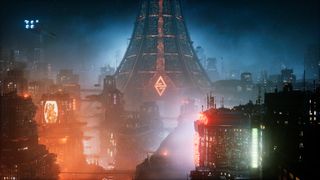This image is a small-sized screen capture seemingly from a CGI-based video game, depicting a futuristic, fictional city enveloped in fog. Dominated by a colossal tower in the background, the actual top of which is cut off, the setting is further shrouded in mystery. The scene is richly detailed, featuring numerous buildings adorned with red, green, and white neon lights that cast a glow through the perpetual night or darkness. This neon illumination gives a sense of liveliness amidst the fog, suggesting a bustling urban environment, albeit one that may be quite polluted. A prominent detail is the number '11' visible in the upper left-hand corner of the image. The taller buildings have intriguing structures, with one particular skyscraper curving upward and marked by a distinctive diamond shape in its middle. The presence of these lights in the windows, though they do not reveal any inhabitants, implies a densely populated city. The overall ambiance hints at an Asian influence without any explicit markers such as writing, enhancing the enigmatic and atmospheric quality of this futuristic landscape.